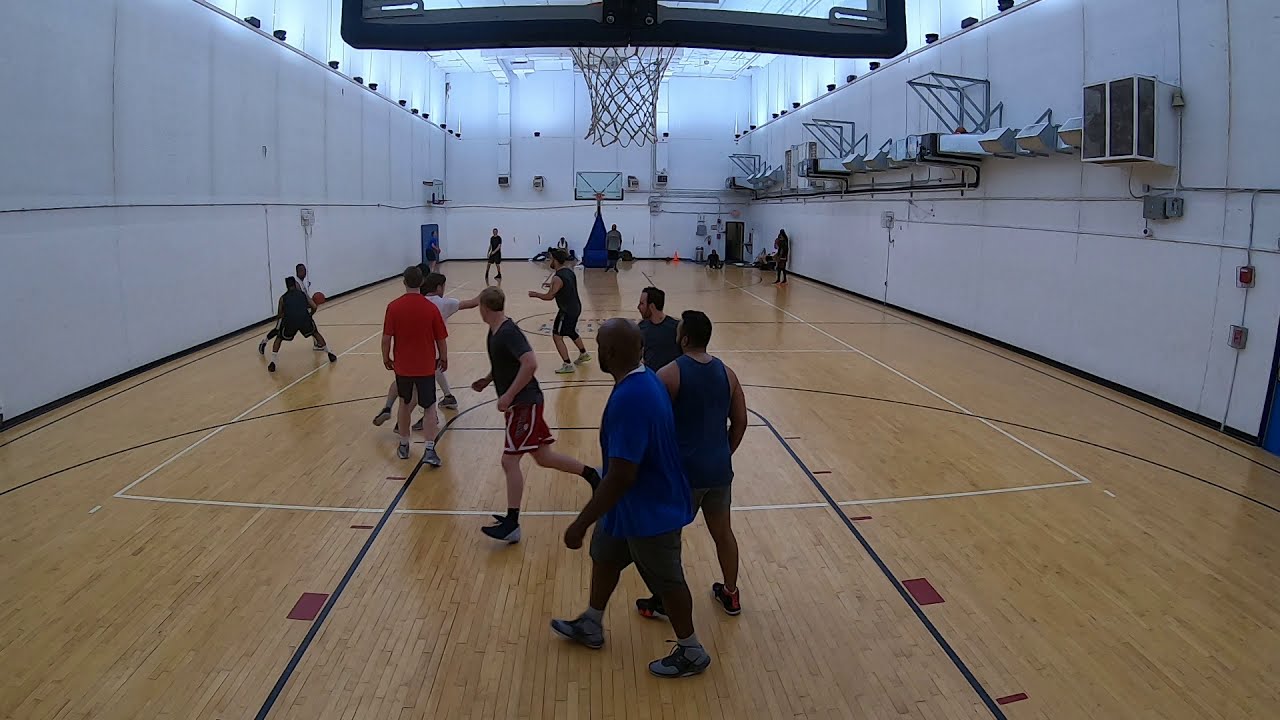This vibrant full-color photograph captures an informal men's basketball game taking place indoors in a gymnasium. The tall white concrete walls of the gym rise high, and the upper third features large windows where light filters through, although no direct sunlight reaches the court itself. The gym floor is wooden and marked with typical basketball court lines. The game is an intramural one, with no official teams or uniforms, showcasing a diverse group of players in terms of age, size, and race.

The image is taken from just behind and slightly below one of the basketball hoops, offering a unique vantage point. Most of the action is near the basket closest to the viewer, where a black player is seen dribbling the ball, attempting to maneuver around an opponent. Nearby, a couple of players are pointing at each other, engaging in animated play. In the background, other participants are dispersed across the full court, adding depth to the scene. The dynamic composition and lively atmosphere highlight the community and casual nature of the game.